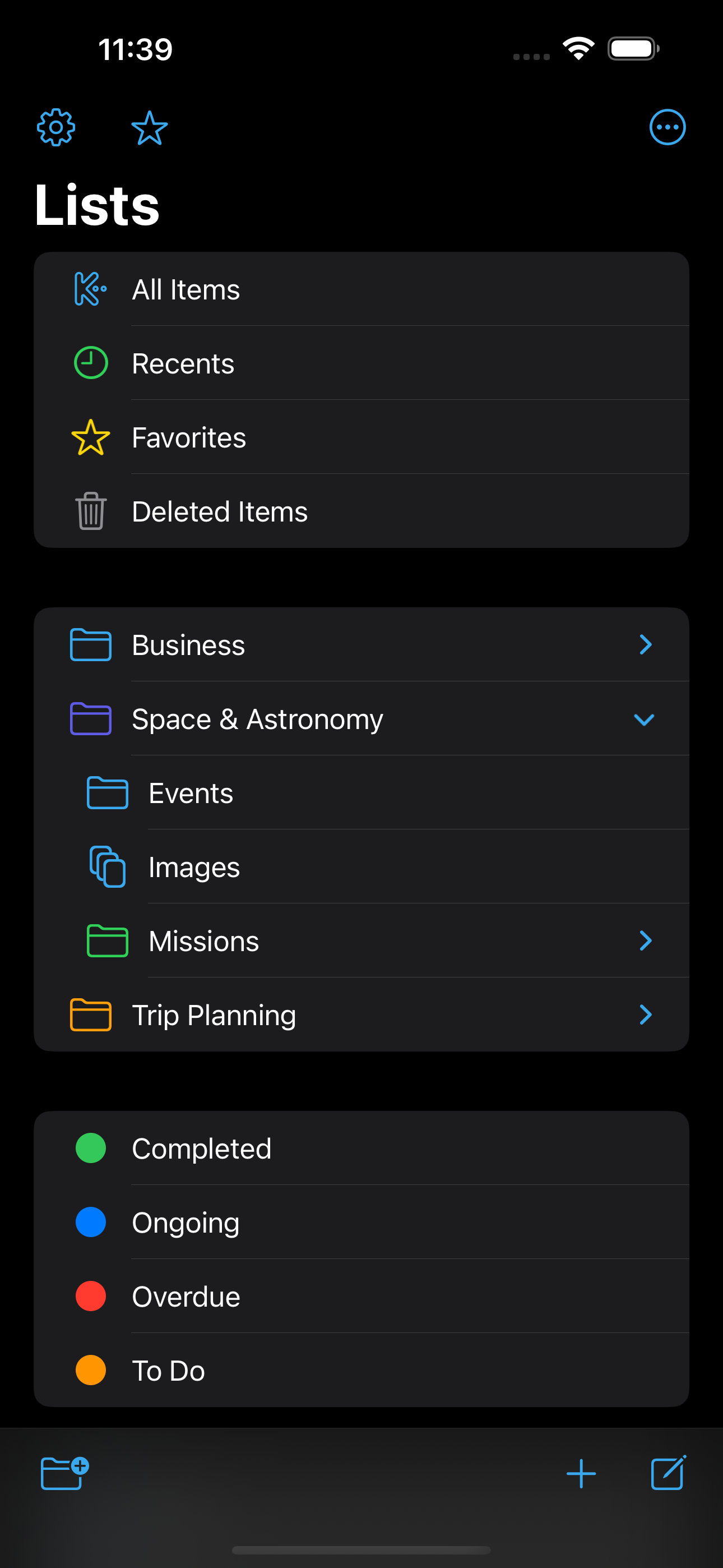This image is a screenshot of a smartphone interface. At the top left, the display shows the network provider name in white text alongside a Wi-Fi icon. Centrally positioned at the top, the time is displayed as 14:38. On the top right, there is a white battery icon indicating a full charge.

Below this status bar, there is a row of icons against a gray background with curved corners. From left to right, these icons include: a blue gear icon for settings, a blue star outline, and a blue circle outline with three blue dots in the center. Adjacent to the blue circle, the word "Lists" appears in white text.

Further down, there is a section featuring four options listed in white text each with an accompanying icon to the left. The options are: "All Items," "Recent," "Favorites," and "Deleted Items."

The subsequent section contains another gray rectangle with curved corners that lists categories and subcategories. It includes "Business," "Space and Astronomy," "Events," "Images," "Missions," and "Trip Planning." Except for "Space and Astronomy," which has an arrow pointing downward indicating expanded content, the other categories have arrows pointing to the right.

Beneath this is a partially visible gray rectangle where "Completed" is displayed next to a green dot, and an incomplete word next to a blue dot.

At the bottom left of the screen, there is a folder icon, and at the bottom right, there is a plus sign and a pencil icon with a small square, likely for adding new items and editing, respectively.

The background of the phone screen is black, enhancing the contrast and visibility of the interface elements.